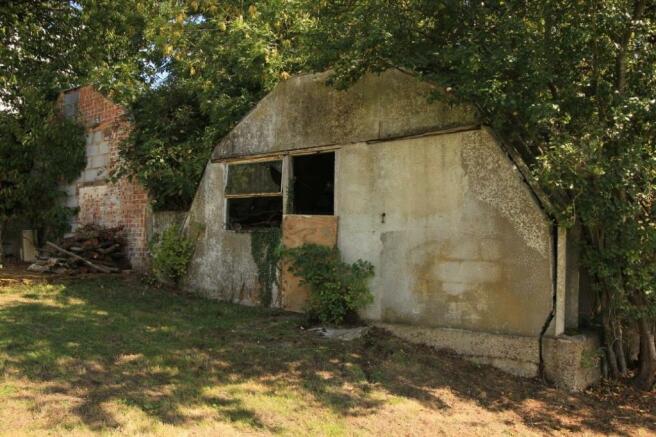In this image, we see an abandoned, arch-shaped old building or shed situated in a wooded area. The structure, which appears to be deteriorating, features a mix of concrete and brick materials. The front of the building showcases a red and white brick wall with a pile of wood stacked at its base, interspersed with cinder blocks. Surrounding this wall are densely packed trees with large green leaves, creating a canopy that partially obscures the building and casts shadows on the ground.

The structure's right side, made of gray concrete, includes two windows. The left window has its bottom half covered with a piece of cardboard, while the right, smaller rectangular window has glass covering just its top half. Both windows and several areas of the building's surface display rust-colored stains, contributing to its neglected appearance. The ground around the building alternates between patches of green grass and brown dirt, with some green shrubs near the building's concrete base. The sky is visible through gaps in the leafy canopy, adding a hint of light to this otherwise somber scene.